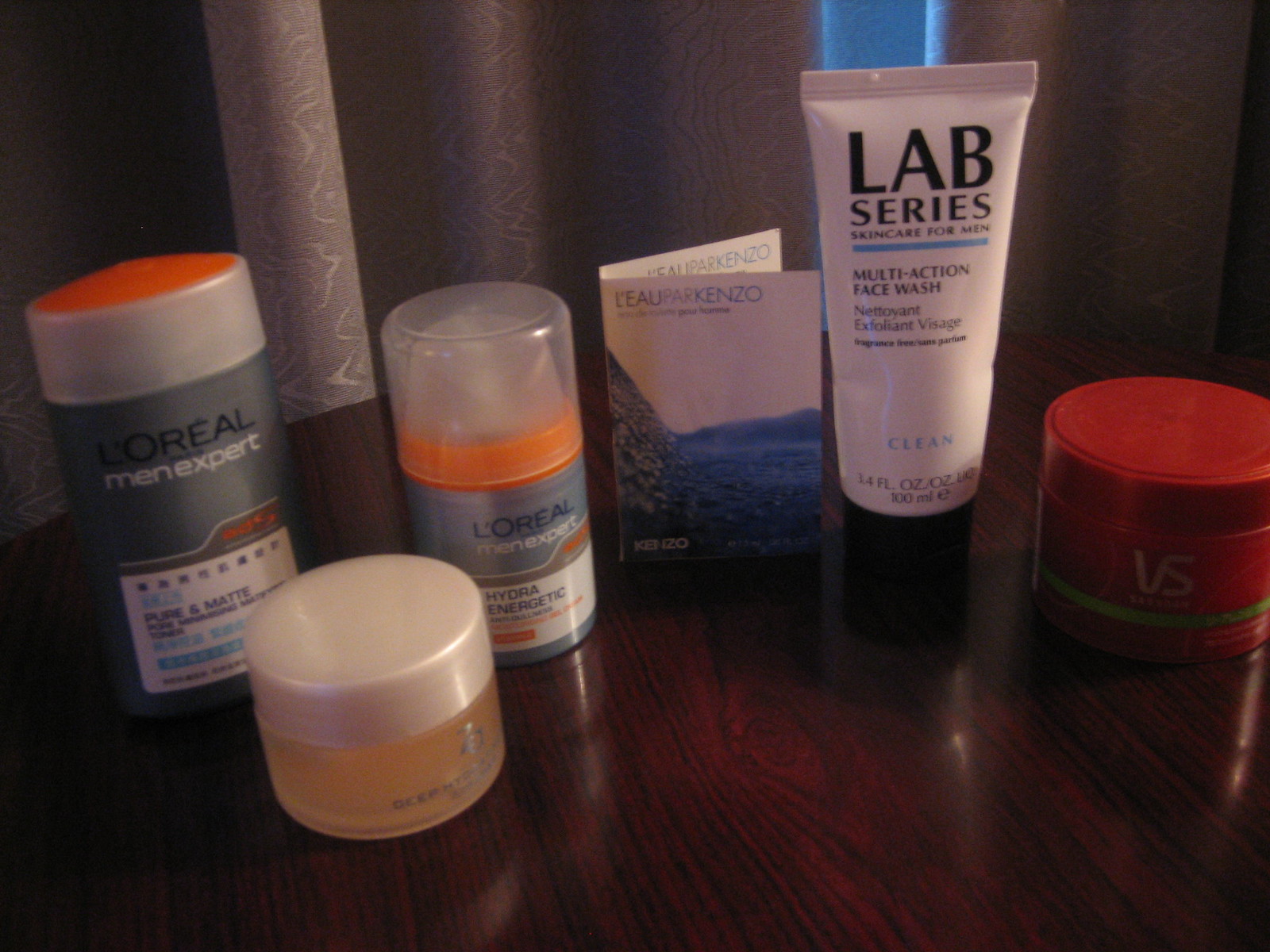The photograph showcases a variety of personal care products arranged on a dark brown wooden table, with the wood grain visibly accentuating the rustic setting. In the background, gray and white patterned curtains add a soft, decorative element to the scene.

On the table, several items are meticulously placed:
1. A cream-colored jar with a white lid.
2. A packaged product in gray, white, black, and blue, labeled "L'Oreal Men Expert Pure and Matte."
3. Another "L'Oreal Men Expert Pure and Matte" product with a white lid.
4. A third "L'Oreal Men Expert Pure and Matte" item, also with a white lid.
5. An additional "L'Oreal Men Expert" product featuring a gray and orange design with a clear lid.
6. A piece of paper with black and blue font, displaying an abstract dirt-like image along with some white text at the bottom.
7. A tube labeled "Lab Series Skin Care for Men," characterized by black font and a white-blue line.
8. Another "L'Oreal Men Expert Pure and Matte" product including a white-blue line and black font, described as a multi-action face wash.
9. The final item on the table is a red and green jar with white font details.

Each product is distinctly presented, offering a comprehensive look at the assortment of men’s skincare products displayed.